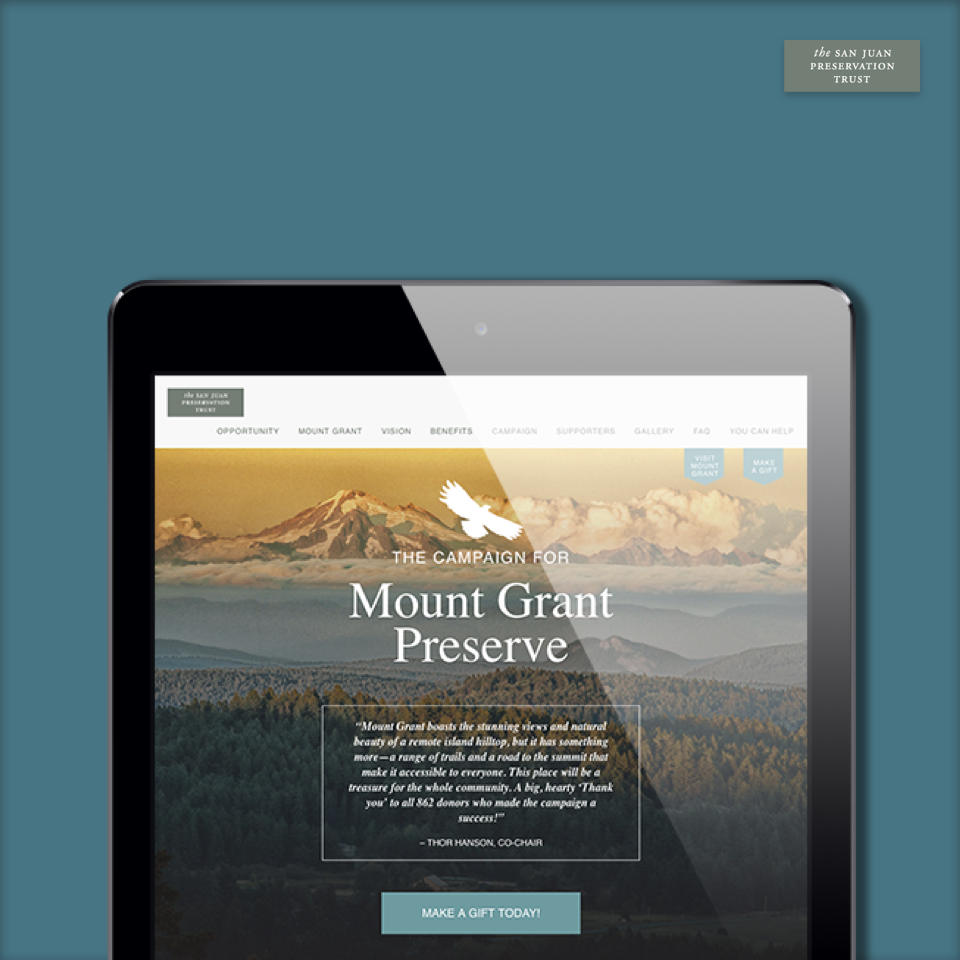In this image, the background transitions through various shades of grey and blue, with the upper right corner featuring a grey box containing white text that reads "The San Juan Preservation Trust." Dominating the center of the image is an iPad with a clear screen. The iPad has a sleek black border, while the screen itself displays content against a white background.

On the left side of the screen, there is a grey column with white lettering, and adjacent to it is a section with black text on a white background. The text line reads sequentially: "Opportunity," "Mount Grant," "Vision," "Benefits," "Campaign," "Supporters Gallery," "FAQ," and "You Can Help." Just below this section are two smaller blocks of text in white font.

At the center of the iPad screen, there is an emblem of a white eagle. Beneath this emblem, in white font, reads the text "The Campaign for Mount Grant Preserve." Directly below this is a white box containing a quote in small white lettering.

The lower part of the image features a light blue box with white text urging "Make a Gift Today." The background of this section showcases grey mountains mingled with white clouds at the bottom. The overall image appears to blend into another scene featuring green trees extending from the foreground towards the mountainous horizon set against an orange sky.